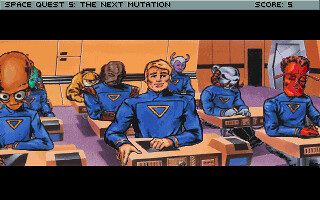The image is a screenshot from the retro point-and-click game "Space Quest V: The Next Mutation," evocative of early 1990s computer games, likely for DOS. The scene depicts a classroom with futuristic yet retro design elements, boasting an orange background and a purple floor. At the top left, the screen displays "SPACE QUEST V: The Next Mutation" along with a score of 5. The classroom is filled with a diverse group of characters, including humans and aliens, all adorned in blue spacesuits. From left to right, there's a large-headed orange alien, a blonde-haired human, a carrot-headed alien, a redhead alien, and a horned alien, all seated at desks. The image is framed by black bars at the top and bottom, giving it the appearance of a paused cinematic sequence within the game.